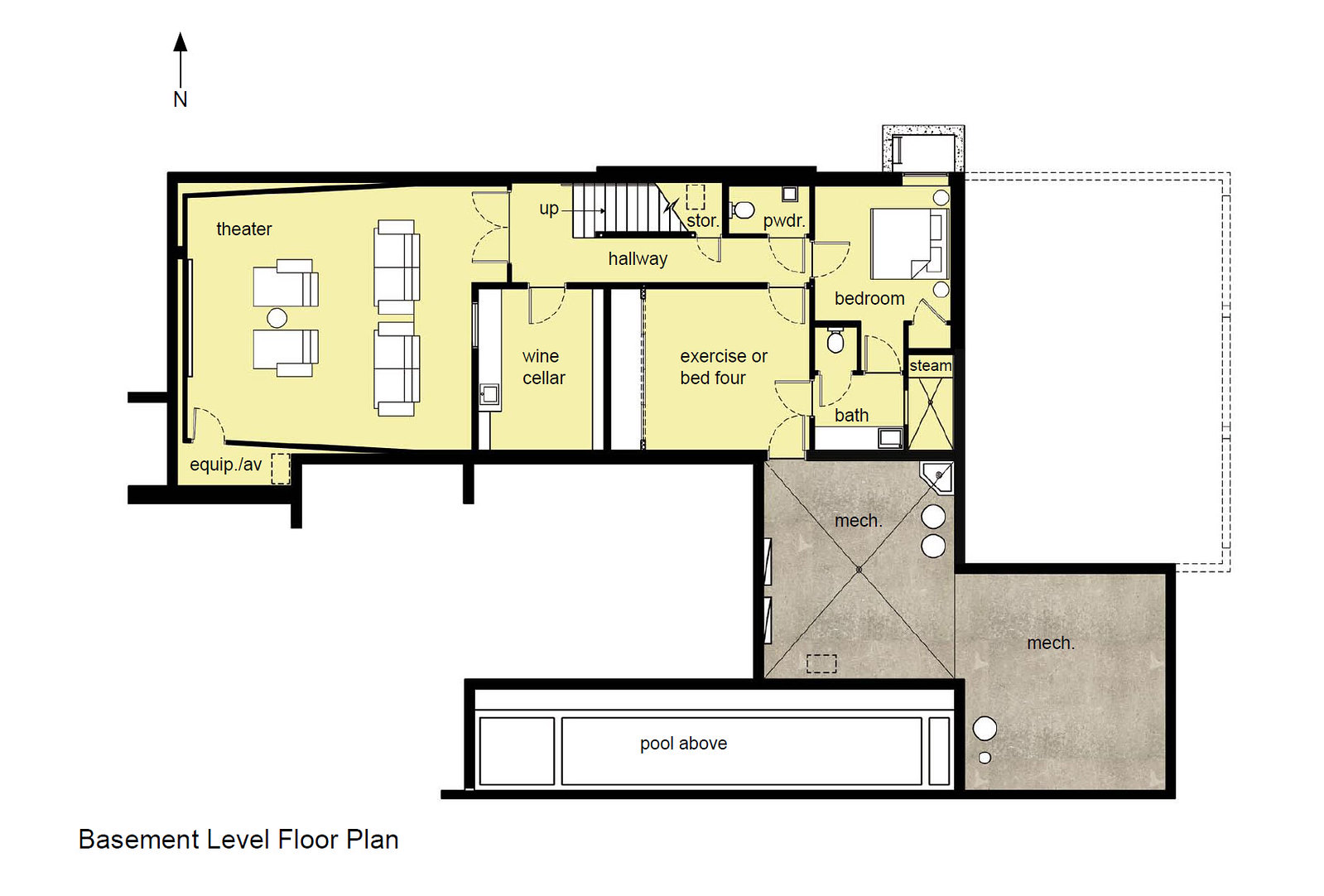This image depicts a detailed floor plan of a basement level, denoted by the text in the bottom left corner. An arrow labeled 'N' at the top left indicates the north direction. The building has an inverted U-shape. On the left side of the plan, a yellow-shaded theater is visible, with white rectangles representing the seating arrangement. Adjacent to the theater, moving inward, are the designated areas for a wine cellar, an exercise room or possibly bedroom 4, and a hallway featuring stairs labeled 'up'. 

The hallway provides access to storage, a powder room, another bedroom, a bathroom, and a steam room, all shaded in yellow with white furnishings depicted within each space. On the right side of the floor plan, a large white rectangle is present, which could indicate an open area or additional room. Below this, two grey squares are labeled as mechanical spaces. At the bottom of the image, three white rectangles encased in a black line depict the pool area, marked 'pool above'. Overall, the plan showcases a well-organized layout of various functional spaces within the basement.